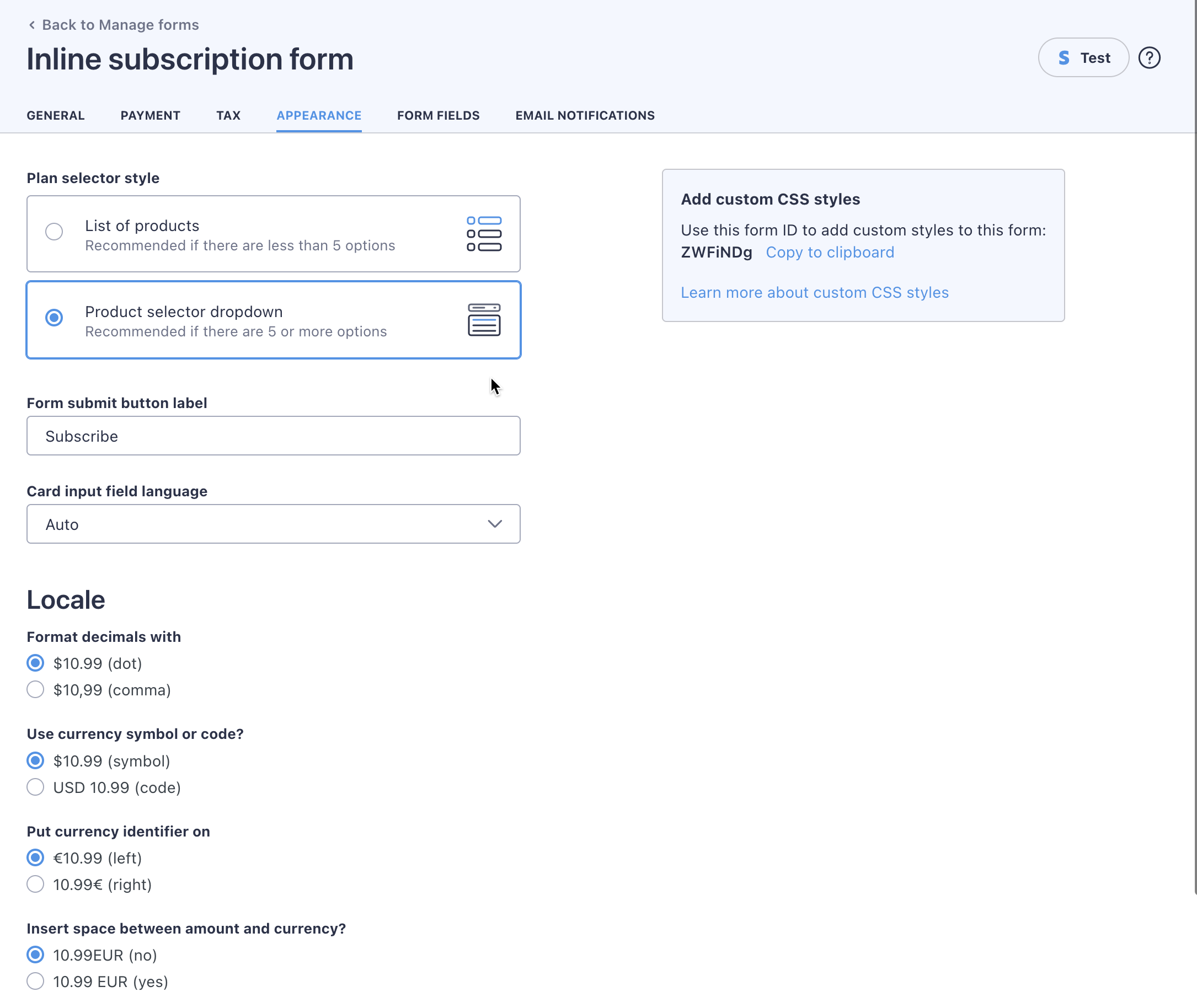Caption: 

The image showcases a user interface for creating a subscription form, set against a pure white background. In the top left corner, the headline "Inline Subscription Form" is prominently displayed. A black text menu at the top lists various configuration options: General, Payment, Tax, Appearance, Form Fields, and Email Notifications. Among these options, "Appearance" is emphasized, underlined in blue, indicating it is currently selected. On the right side, there is an option to "Add Custom CSS Styles," with a feature to copy styles to the clipboard. A "Test" button is also visible, suggesting a tool to preview the form's functionality. A gray bar runs along the far right side, providing additional navigation, and at the top of the interface, a link labeled "Back to Manage Forms" allows users to return to previous tasks. The clean, minimalistic design ensures clarity and ease of use for custom form creation.